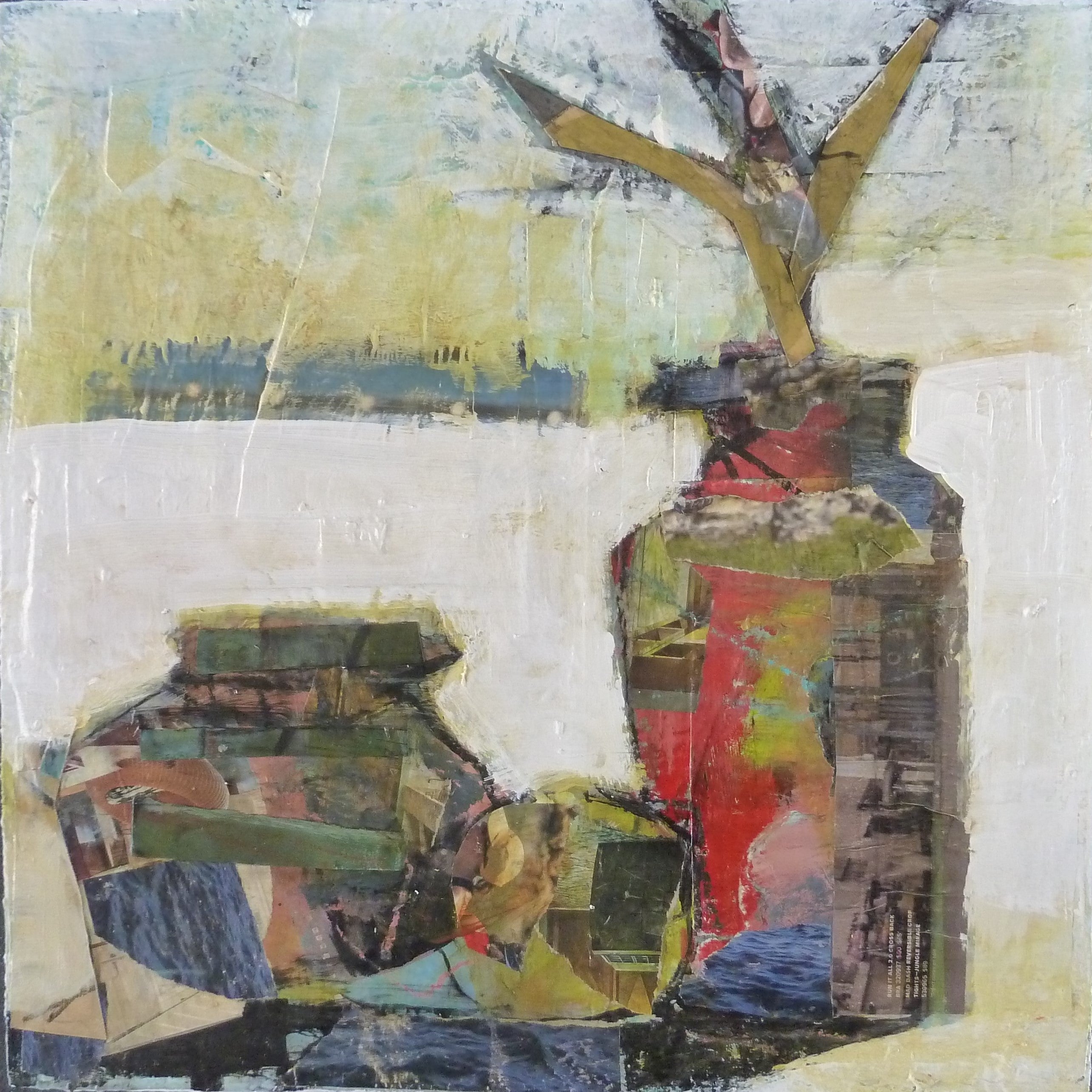The painting depicted in the image is a vibrant yet abstract composition, likely created with acrylics. It features a large vertical structure resembling a flower pot or vase made from a collage of reds, blacks, and other hues, incorporating elements that appear to be cut from newspapers or magazines. Above it, there are three branch-like extensions, contributing to the overall impression of a plant. To the right, another rounded object, potentially a teapot, and a yellow shape add to the complex imagery.

Despite its bright and varied colors, including red, green, blue, black, white, and beige, the painting has a muted, aged look, as if faded over time. The background features white and greenish-blue elements, possibly suggesting a fence or horizon with a train-like shape faintly visible on it. The entire scene is rendered in a Cubist-inspired style, blending shapes and colors into an elusive, almost dreamlike abstraction. The image is well-lit, revealing the intricate details and textured brushstrokes that create this rich and enigmatic work of art.